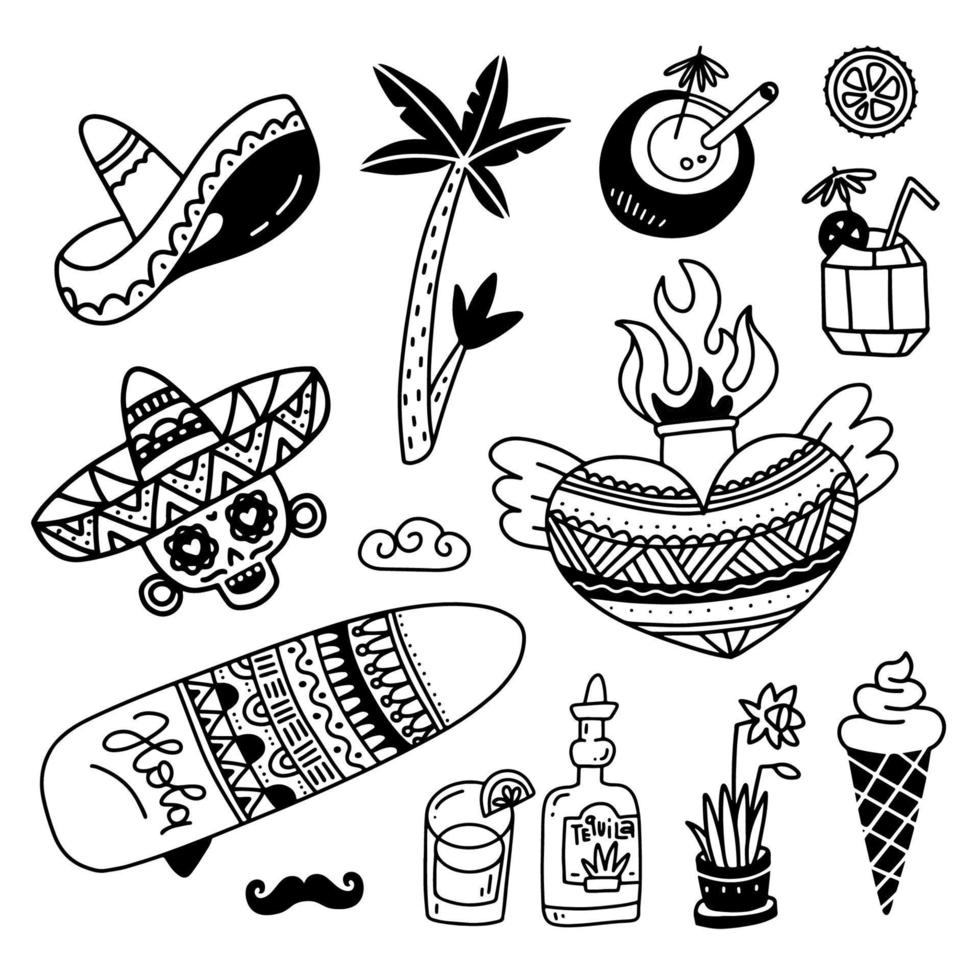The image is a black and white illustration with various Mexican-themed elements spread across it. Dominating the center is a giant heart pot with wings and flames erupting from its top. Towards the center-left area, a palm tree is visible, adding a tropical touch. On the top right corner, there's a slice of orange. The right side of the image features multiple items: a sombrero and a skull wearing a sombrero, positioned above a large object that has "Hola" written repeatedly along its bottom edge. Directly below the skull and sombrero is a random mustache. To the right of the mustache is a glass with a drink garnished with a lemon wedge, followed by a tequila bottle, a flower pot, and an ice cream cone in that order. The overall scene is decorated with line drawings, embodying themes typical of Dia de los Muertos, including spirited motifs and intricate designs reminiscent of Mayan or Aztec art.